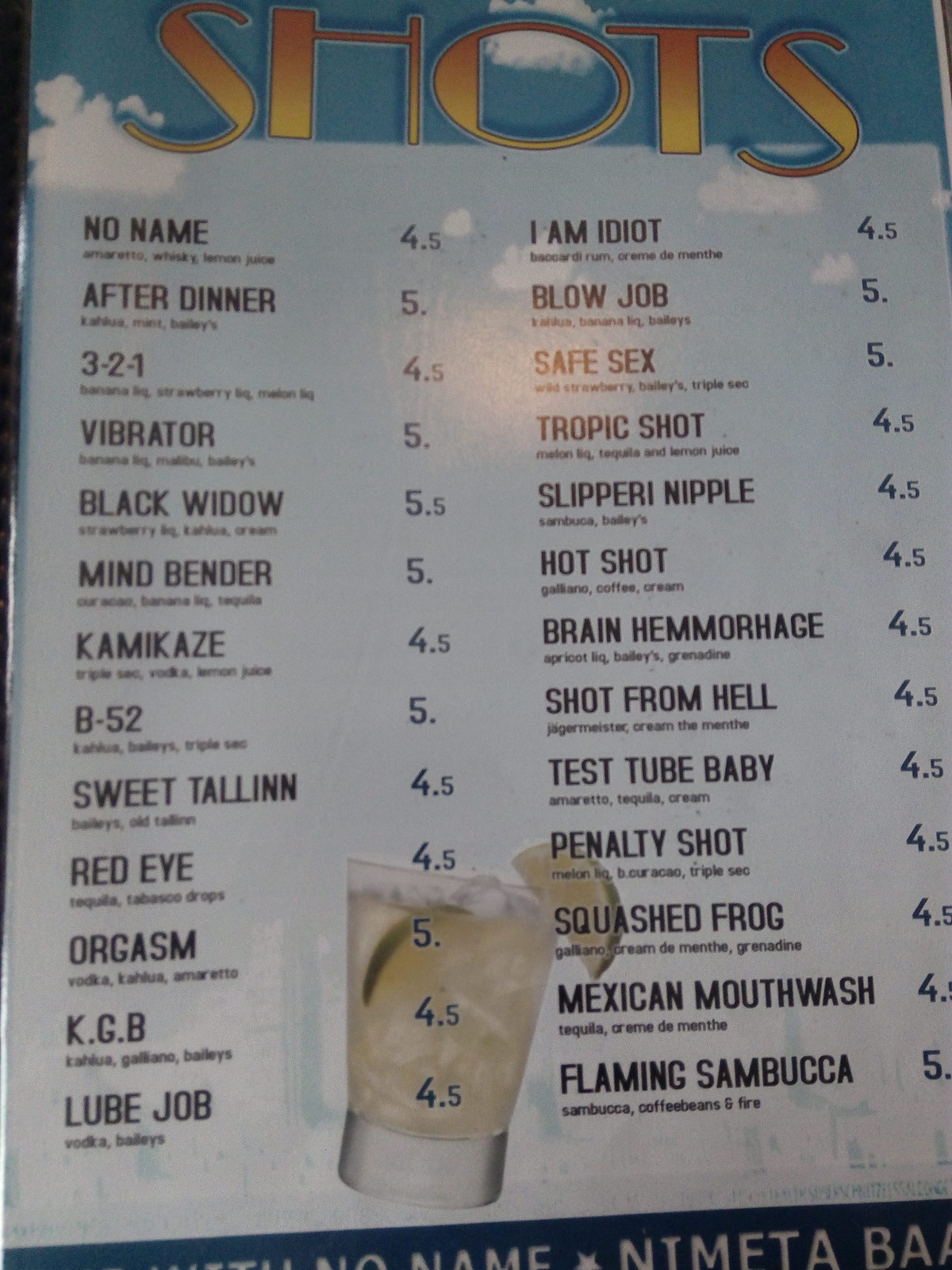The image is a colorful menu showcasing various alcoholic shots against a sky-themed background with blue hues and white clouds. At the top, the word "Shots" is prominently displayed in bold, yellow bubble letters. The left side of the menu lists shot names in black text, starting with "No Name" priced at 4, followed by "After Dinner," "3 2 1," "Vibrator," "Black Widow," "Mind Bender," "Kamikaze," "B-52," "Sweet Tollen," "Red-Eye," "Orgasm," "KGB," and "Lube Job." An accompanying image features a vibrant yellow shot garnished with a lime wedge on the rim and a lime piece inside the glass.

On the right side, the menu continues with additional shot names, starting from the top: "I Am Idiot," "Blowjob," "Safe Sex," "Tropic Shot," "Slippery Nipple," "Hot Shot," "Brain Hemorrhage," "Shot from Hell," "Test Tube Baby," "Penalty Shot," "Squashed Frog," "Mexican Mouthwash," and "Flaming Sambuca." Most of these shots are priced at 4.5, with a few marked at 5. At the bottom of the menu, there is additional text that reads "NTM ETA BA," although its significance is unclear.